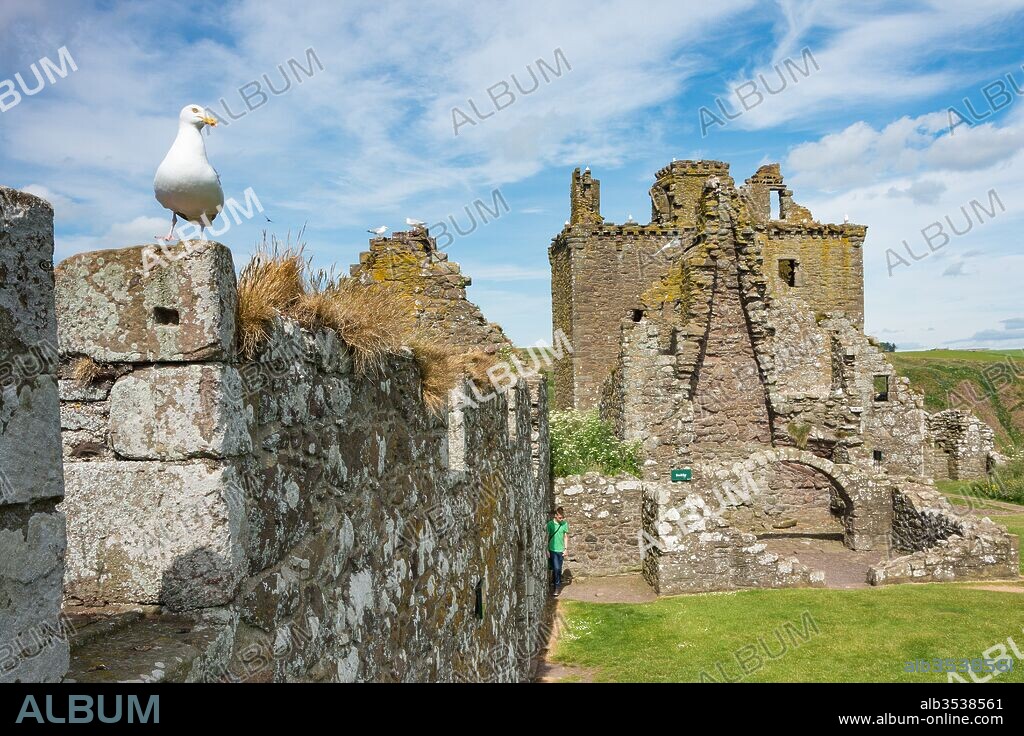The color photograph shows the picturesque ruins of an old stone castle somewhere in the UK, bathed in natural sunlight under a blue sky dotted with white clouds. At the forefront on the left side, a seagull perches atop a jagged stone wall, with more gulls scattered across different parts of the ruin’s roof. The main structure on the right features an irregular, weathered stone architecture, punctuated by a stone archway that once served as an entrance and traces of windows and a chimney. A person wearing a green shirt and blue pants can be seen walking along a grassy path near the base of the ruins. The entire scene is overlaid with about 10 to 15 watermarks reading "album," and a black border at the bottom features the text "ALBUM" on the left and "ALB 353 8561 www.album-online.com" on the right.